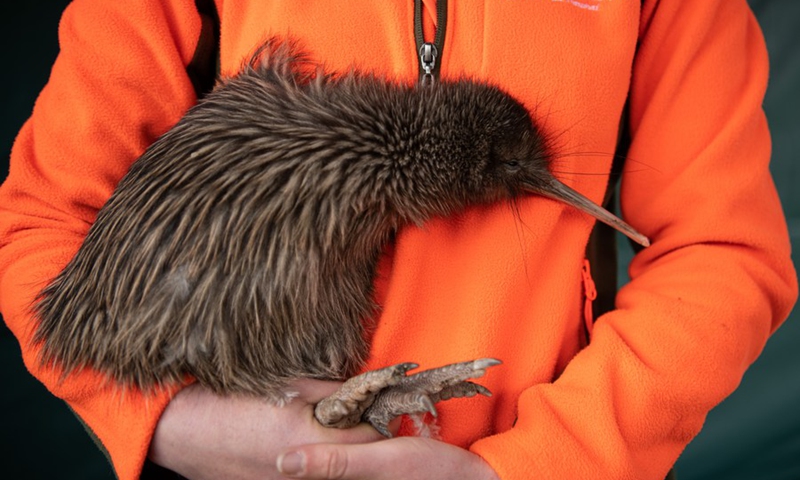In this portrait-oriented photograph, a person dressed in an orange long-sleeve jacket with a centered zipper and a pocket on the left side cradles a large bird against their chest. The person, who appears to have light skin, is holding the bird with both hands at the bottom of the image. The backdrop is black, enhancing the vividness of the orange jacket. The bird, likely a duck, is predominantly brown with a gradient of feather colors transitioning from dark brown to lighter shades, and has fluffy, almost fur-like feathers with small patches of white. Its long, thin, pointy beak is dark brown or black, and it has a partially closed, sleepy-looking brown eye. The bird’s talons are light tan to light gray and appear very sharp. The scene portrays the bird looking somewhat scared, confused, or disoriented.